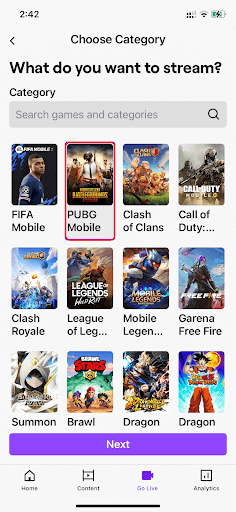This image captures a screenshot of a mobile phone display set against a pristine white background. The top-left corner shows the current time, 2:42, while the upper right corner features standard icons, including reception bars, Wi-Fi signal, and battery level. Just below these indicators is a navigation element labeled "Choose Category" accompanied by a left-pointing arrow. 

Dominating the center of the screen is a bold black text headline that reads, "What do you want to stream?" Directly underneath, there is a grey search box that invites users to "Search games and categories."

The screen is segmented into two distinct rows of game titles. The first row begins with "FIFA Mobile" on the far left, followed by "PUBG Mobile," which is outlined in red, then "Clash of Clans," and ending with "Call of Duty." The second row starts with "Clash Royale" and continues with "League of Legends," "Mobile Legends," and concludes with "Garena Free Fire" on the far right.

Each game title is clearly separated from the others, creating an organized and user-friendly interface for browsing streaming options.